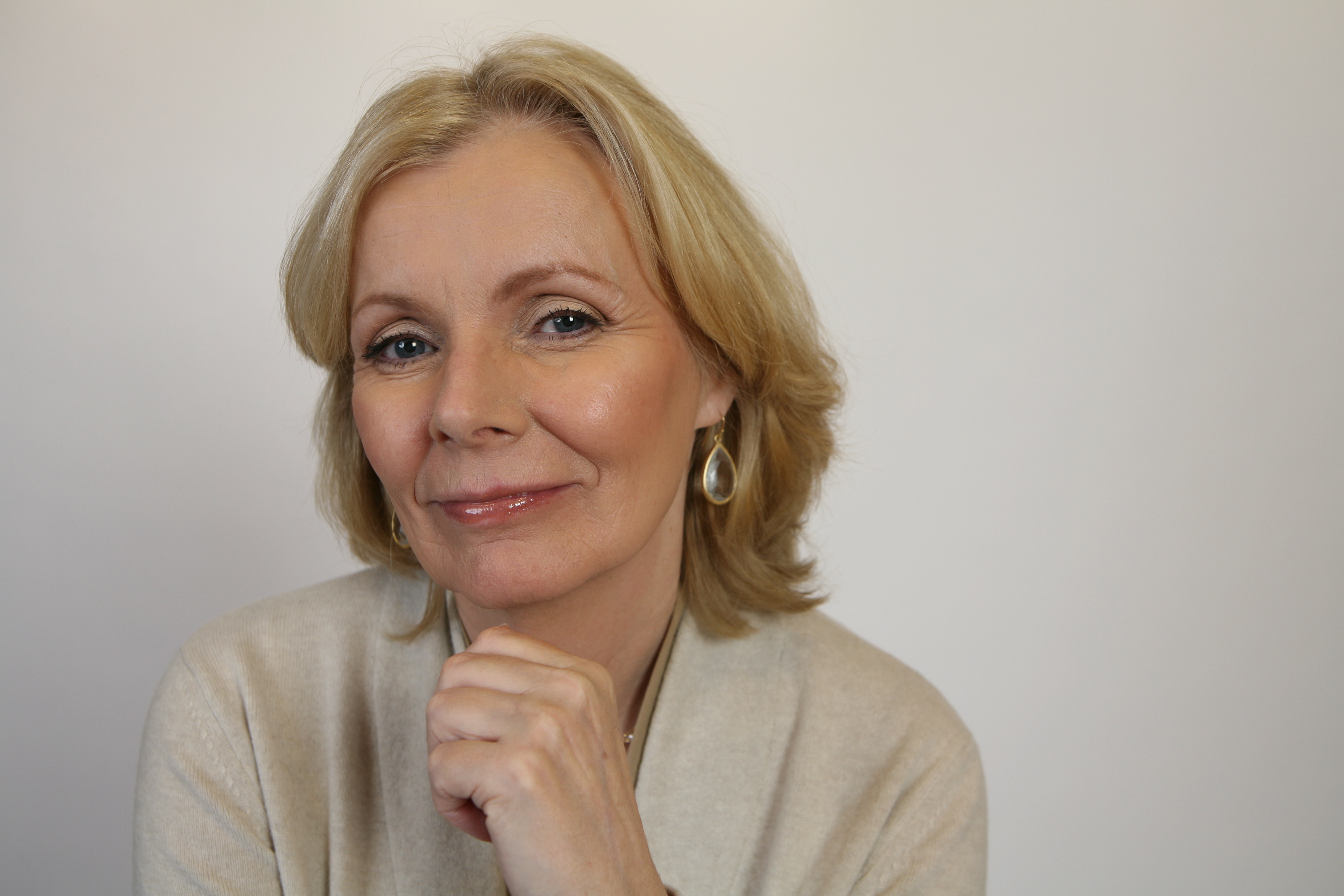The photograph depicts an older woman, likely in her 50s or 60s, positioned slightly to the left of the frame. She has shoulder-length, wavy blonde hair and green eyes, highlighted by red lipstick and a smile. Her complexion is fair, and her glossy lips suggest well-maintained skin. She wears a white or beige top, with faint hints of a green garment underneath, though this detail is subtle. Her left hand is gently resting under her chin, with fingers balled into a fist. She accessorizes with dangly earrings that appear to be a mix of black, gold, and beige colors with oval shapes. The background features a gradient, transitioning from a bright white at the top to a grayer tone towards the bottom and edges, creating a neutral and soft ambiance.